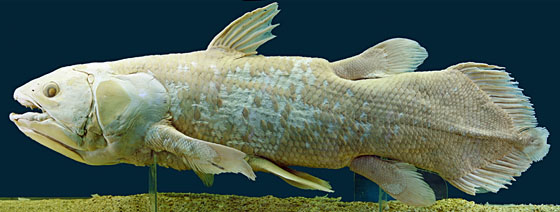This image showcases a mounted coelacanth, a fish once thought to be extinct, displayed in a long, narrow, rectangular photograph. The background is predominantly black, fading slightly in areas to give a lit effect. The fish itself lies on green and tan gravel, suggesting a seafloor scene, and is supported by clear mounts.

The coelacanth's body features tan and white scales, with some areas exhibiting a greenish-gray tint. It has a substantial tail spread out to the back and exhibits various fins along its midsection and near the tail. The fish's jagged gills are visible, and its mouth is slightly agape, hinting at an aggressive nature. The top of the fish's head is predominantly white, and its dark, tan-tinted eye is easily noticeable. The photograph captures the intricate details of the fish's preserved state, highlighting its historical significance.